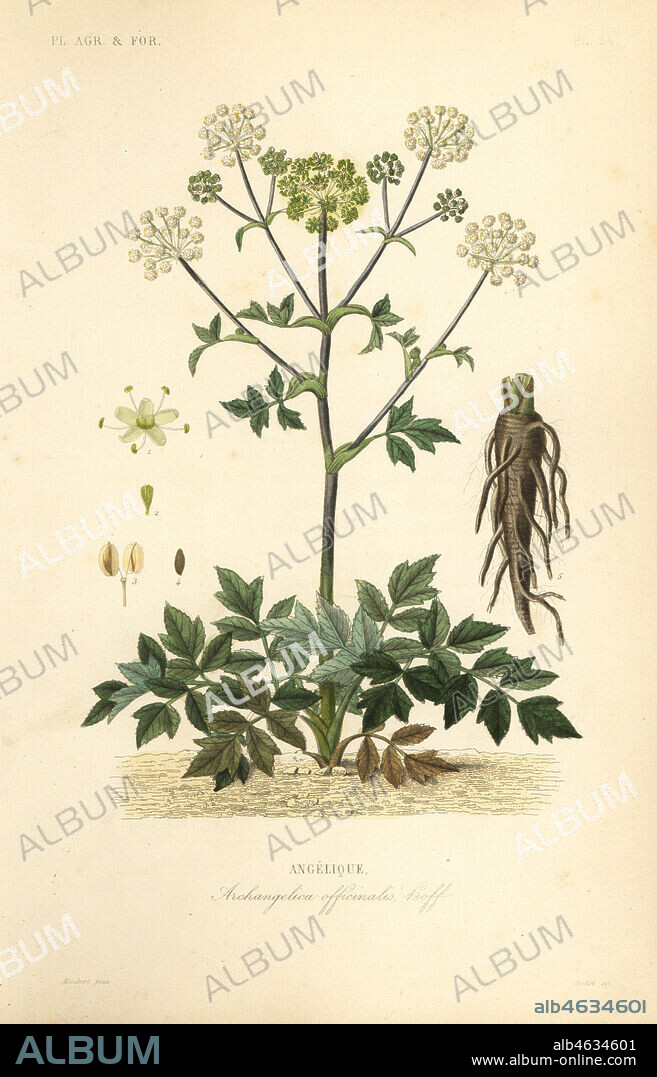The image appears to be a detailed, light-peach or tan-background scientific drawing, most likely a botanical study of a plant. Dominated by the text “FL AGR and FOR” at the top, the image features a central illustration of a plant with most of its leaves concentrated at the base. The plant has a long stem extending upward, culminating in several clusters of mostly white flowers that resemble buds or dill. To the left of the main plant, there is a detailed close-up of the flowers showcasing their intricate pistils, and illustrations of seeds and seed pods. On the right side, the root system is depicted prominently. At the very bottom, the words "Angelique" and possibly "Archangelica/Archangelion" are inscribed. Across the entire image is a gray, uppercase watermark that repetitively states "album." A black border at the bottom contains blue text reading "album" and a reference number "ALB 4634601," along with the URL "www.album-online.com."